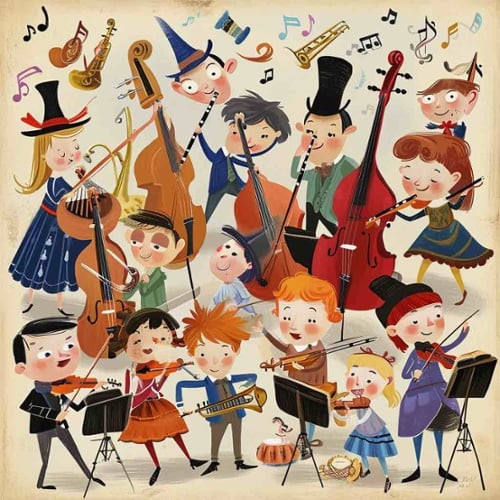This vibrant cartoon-like drawing depicts a lively ensemble of around 14 characters, predominantly children, all playing various musical instruments. In the front row, five children are enthusiastically engaged in their music, equipped with sheet music on stands. Among them, a boy in the lower left corner plays a violin, while to his right, a red-haired boy appears to be playing a trumpet. The children are dressed warmly, suggesting a cold setting. Behind them is a second row with more children and a mix of older children or adults, showcasing woodwind instruments and multiple violins. Notably, a girl in a blue dress plays a cello, and beside her stands a boy holding a clarinet. The highest part of the image features floating instruments, colorful musical notes, and even a whimsical head with a witch-like hat, adding to the unique and crowded composition. The background is a pale beige, and the characters, with their rosy cheeks and tiny feet, are overlapped, ensuring no part of the image is left unfilled. Each character is depicted vividly—a girl in a black hat and blue dress plays the violin on the top left, a boy in blue and gray tackles the bass guitar to the right, and a girl with red hair in a blue dress plays the flute on the far right. The amalgamation of instruments, characters, and musical notes creates an energetic and densely packed illustration of a joyful musical gathering.